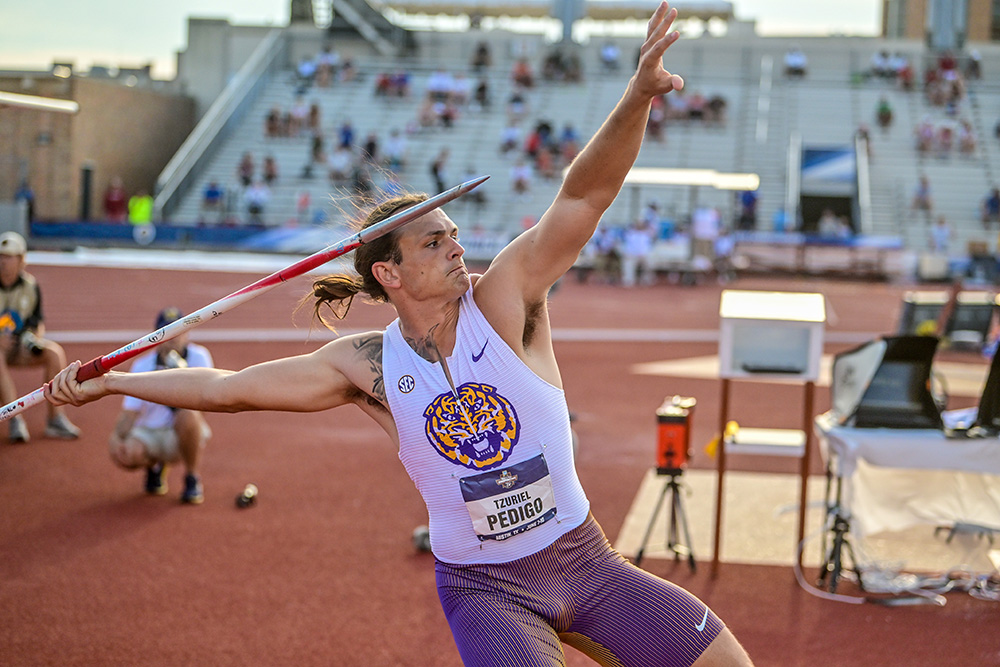In this action-packed photograph taken at an outdoor track and field event, we see a male college athlete from LSU, focused and poised to throw a javelin. The image captures him in mid-motion, leaning back, with the javelin gripped in his hand, ready for release. He is clad in a white sleeveless top featuring the LSU Tigers logo and vibrant purple Nike Lycra compression shorts that end above his thighs. His long brown hair is tied back in a ponytail, and a hint of a tattoo peeks out from his right shoulder under his shirt. The javelin he holds has a distinctive candy cane-like red and white swirl pattern.

In the foreground, where the athlete stands on a brownish-orange terracotta track, the image maintains sharp focus, while the background blends into a softer blur. Behind him, a modest crowd of spectators is scattered across bleachers, watching the competition intently. Nearby, a table with various equipment is set up, possibly for the athletes or judges. A man is crouched down, watching the athlete closely, while another official sits in a chair, looking in a different direction. The image, with its dynamic composition and slight motion blur, effectively captures the tension and excitement of the moment.